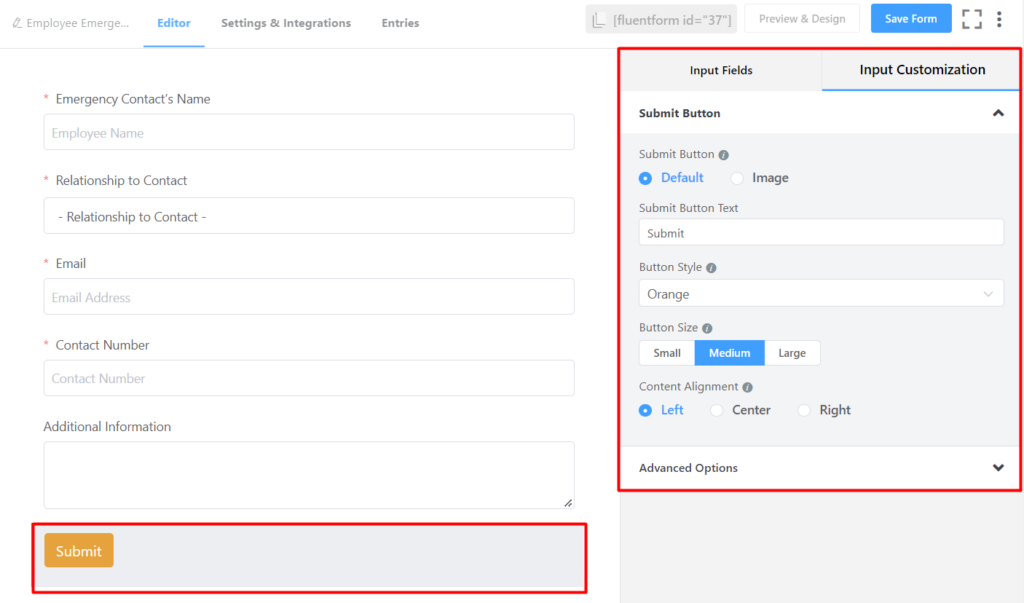This image displays the interface of an employee management system, specifically focusing on the "Employee Emergency Editor" section. The page includes various settings and integrations, allowing users to manage relationships to contacts, input email addresses, contact numbers, and add additional information. Key interactive elements such as "Submit," "Save Form," and options for input customization, including different input fields, are clearly visible.

Towards the bottom of the form, there are size settings (Small, Medium, Large) and alignment options (Left, Center, Right) for an embedded image. Notably, the "Submit" button and the right settings pane are highlighted with red bars, drawing attention to these critical areas.